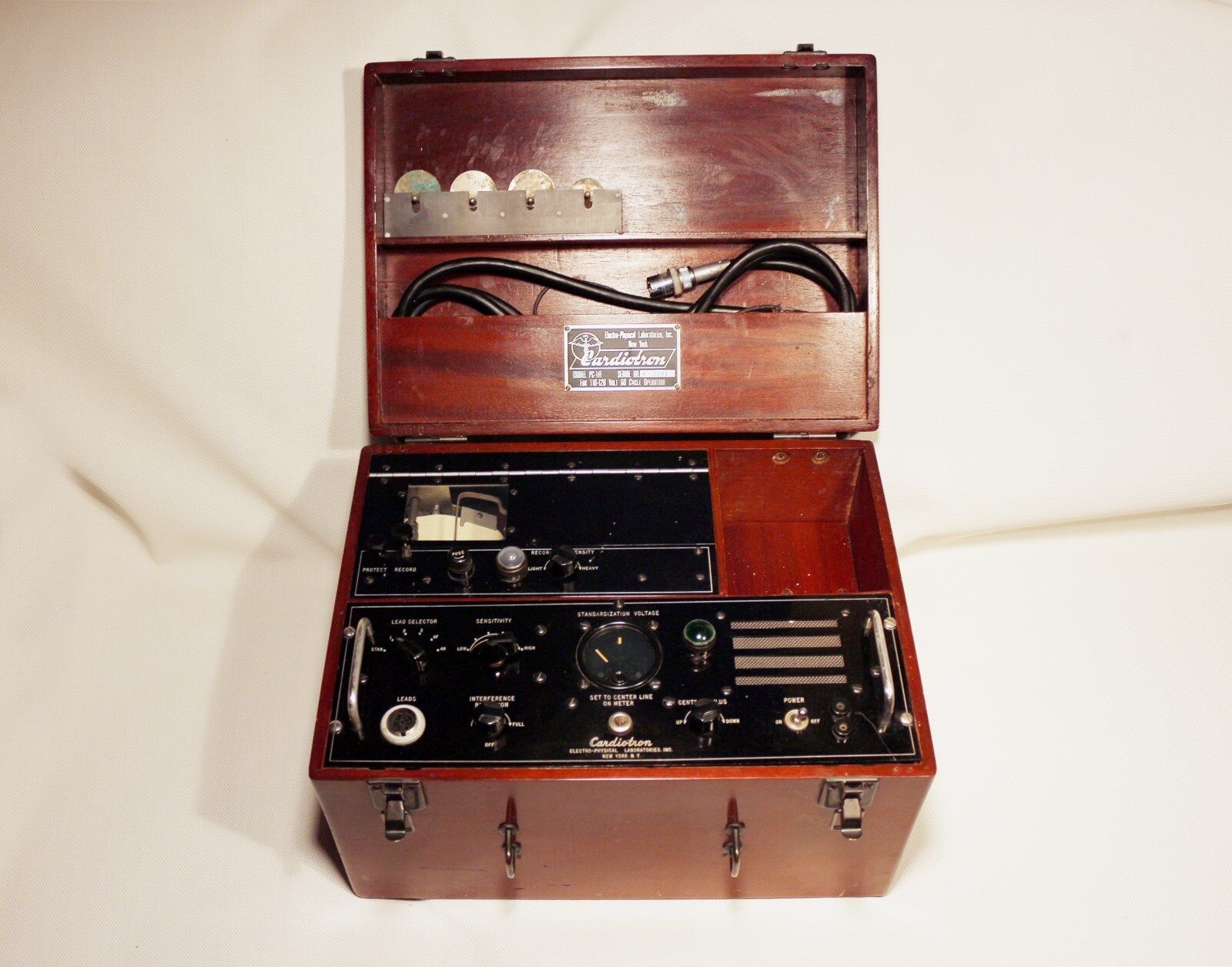The image depicts an antique device housed in a polished, reddish-brown wooden carrying case, set against a white, creased cloth background, likely staged for a sale listing. The box resembles a vintage piece, possibly from the 1950s or 60s, and opens to reveal a sophisticated interior. Inside the lid, which is propped open, there are several compartments holding a cord and small silver discs, likely components of the device. The main section of the case contains two large black units adorned with numerous gauges, dials, and calibration options. Despite the intricate hardware, the precise function of the device remains unclear, though it could be related to quack medicine, possibly using methods like auditory stimulation or electricity. A metal plaque inside suggests the manufacturer’s name, adding historical and possibly collectible value to the equipment.